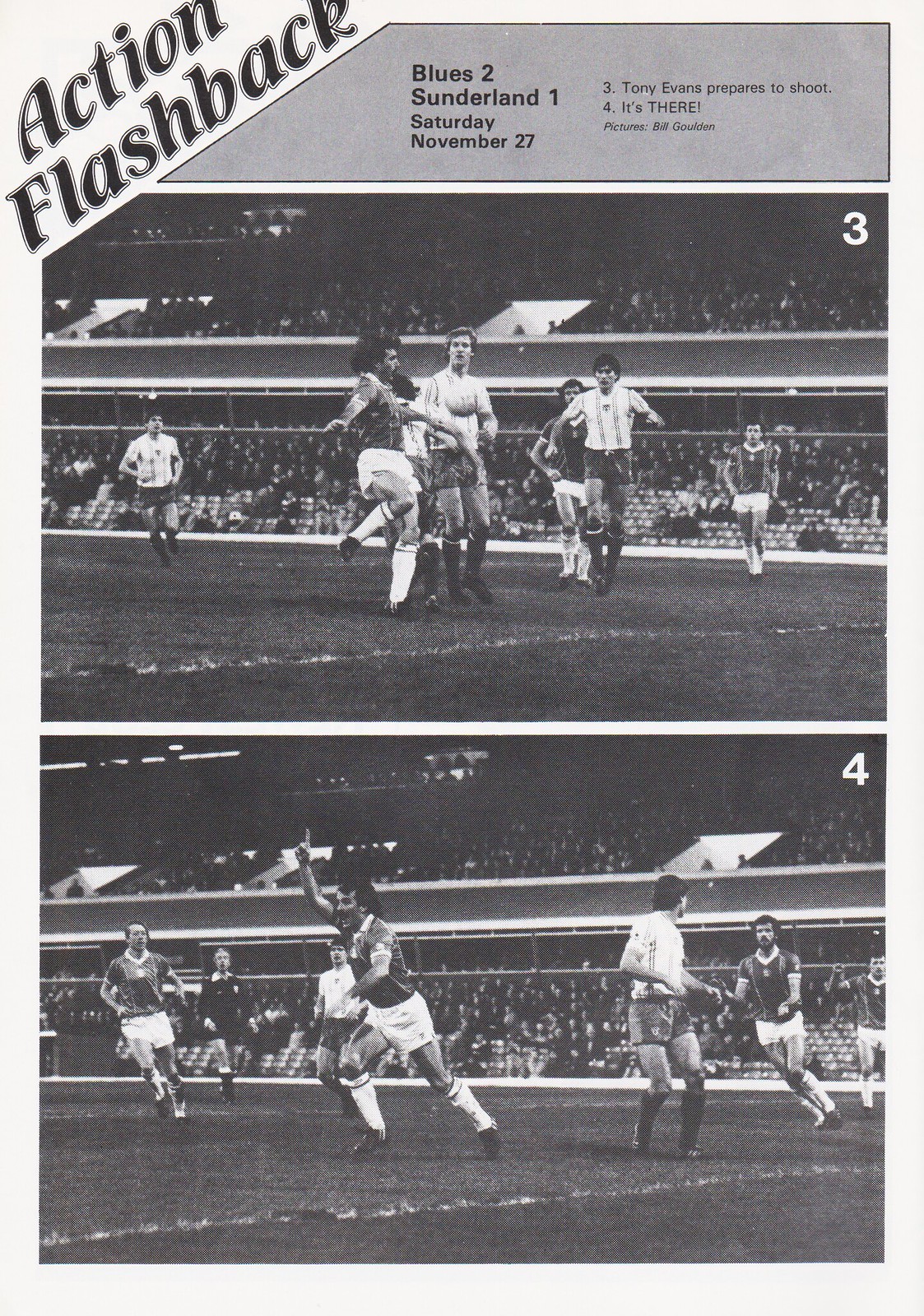This black-and-white image captures the thrilling moments of a soccer match, documented on the cover of a vintage sports program titled "Action Flashback." The top left corner prominently displays the words "Action Flashback," indicating a nostalgic recount of a past game. Below this, a gray bar contains the details: "Blues 2, Sunderland 1, Saturday, November 27th," marking the score and date of the match.

The page features two black-and-white photographs, one above the other, each numbered in the corner. The top photograph, labeled with a "3" in the upper right corner, depicts several soccer players on an athletic field. One player, identified as Tony Evans, is captured mid-action, preparing to shoot the ball. His leg is raised, indicating movement, while other players in white jerseys converge towards him.

Below this, the second photograph is labeled with a "4" in the lower right corner. It seizes the victorious moment right after the successful goal; Tony Evans is seen celebrating with his hands raised high, a smile on his face. His elated teammates rush towards him, ready to congratulate. The background of both photographs shows stands packed with spectators, emphasizing the significance and electric atmosphere of the match.